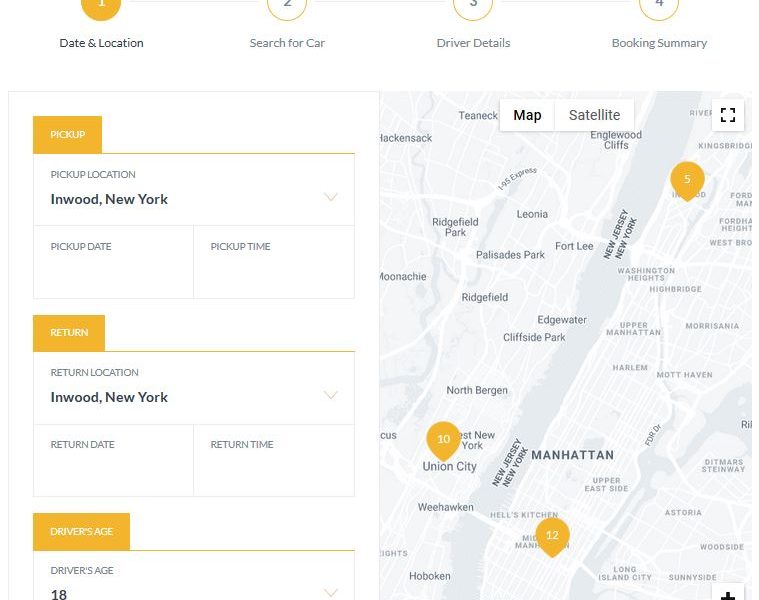The image features a user interface for a car booking platform divided into several sections:

1. **Step Indicator at the Top**:
   - **Round Icon with Number 1**: Orange in color, labeled "Date and Location."
   - **Round Icon with Number 2**: White in color, labeled "Search for Car."
   - **Round Icon with Number 3**: White in color, labeled "Driver Details."
   - **Round Icon with Number 4**: White in color, labeled "Booking Summary."

2. **Pickup Information Section**:
   - **Left Side**:
     - **Orange Button**: Labeled "Pick Up."
     - **Text Fields**: 
       - "Pick Up Location: Inwood, New York."
       - "Pick Up Date"
       - "Pick Up Time"
     
3. **Return Information Section**:
   - **Left Side**:
     - **Orange Button**: Labeled "Return."
     - **Text Fields**:
       - "Return Location: Inwood, New York."
       - "Return Date"
       - "Return Time"
   
4. **Driver Information Section**:
   - **Left Side**:
     - **Orange Box**: Labeled "Driver's Age."
     - **Text Field**: 
       - "Driver's Age: 18."

5. **Map Section**:
   - **Right Side**: A map of Manhattan and the New York City area is displayed, highlighting three push pins:
     - **Push Pin in the Bronx.**
     - **Push Pin in Union City, New Jersey.**
     - **Push Pin in Downtown Manhattan.**

This layout provides clear, step-by-step guidance for booking a car, with specific locations, dates, times, and driver's age details required for the reservation, and includes a map for visual reference of pertinent locations.